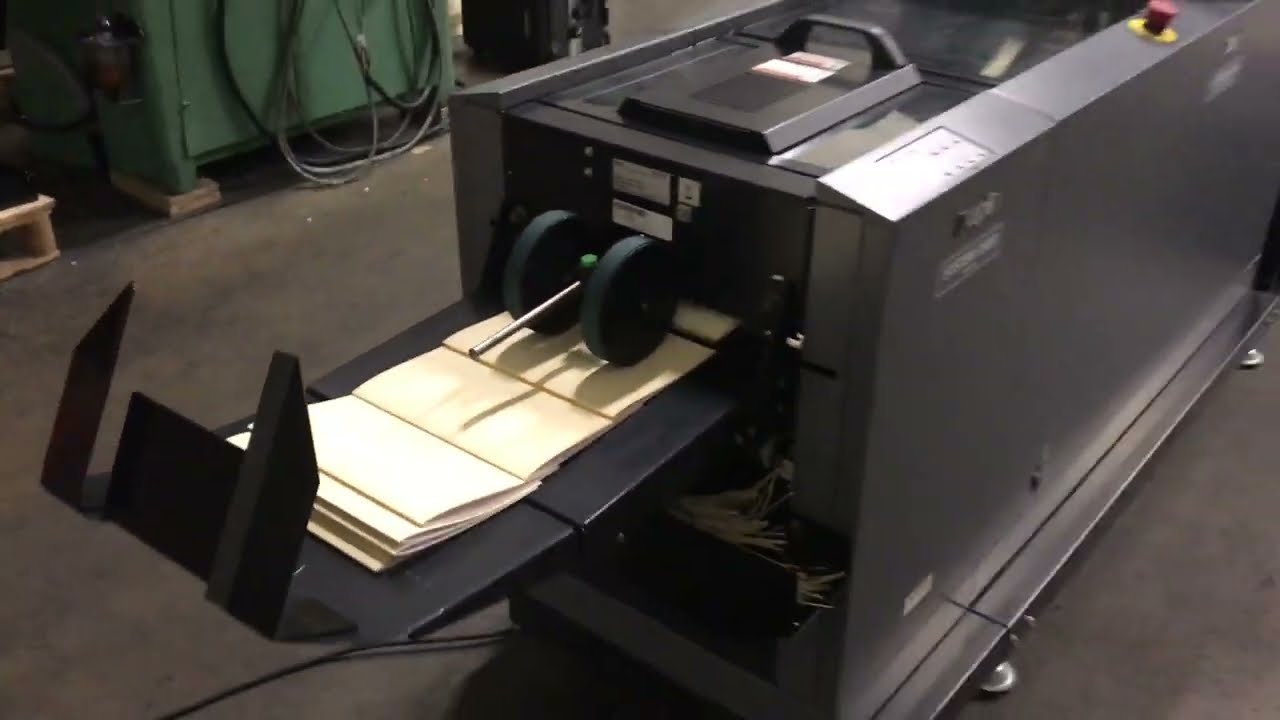The image depicts an industrial scene featuring a steel rectangular machine, likely involved in the production of pamphlets, situated on a concrete floor in a factory environment. The main focus is the silver-gray machine in the foreground, characterized by a prominent red emergency stop button on its top middle section. Attached to this machine is a feeder tray with several black compartments, possibly designed to hold and organize the output. Black square trays or pegs with flat ends extend from the feeder, guiding the pamphlets that the machine produces.

Papers, tan in color and folded, rest on the machine, indicative of the machine's folding function. A pair of round wheels with a slender silver rod between them appears on these papers, likely part of the mechanism that guides or processes them. In the output tray, multiple pamphlets or envelopes are actively being dispensed, suggesting a continuous operation. Beneath this machine, a bin holds white shredded paper, likely the trimmed excess from the pamphlets.

The background features another green machine adorned with looping hoses, reinforcing the industrial setting. The floor shows signs of wear and dirt, typical of a factory, while the walls and other equipment, such as the green machine, maintain a utilitarian and functional appearance.